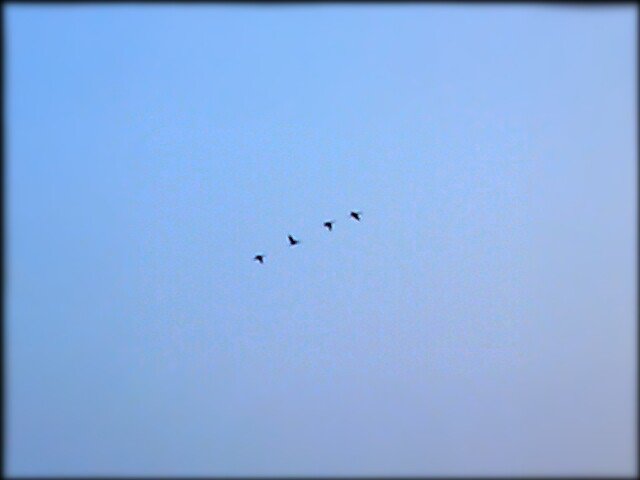This image captures a clear, light blue sky devoid of clouds, with four small, dark birds flying in the distance. Despite their size and the altitude of their flight, their long wings are discernible. They are aligned in an ascending oblique line, facing the upper right-hand corner of the rectangular, landscape-oriented photo. Each bird is equidistant from the next, with their wing positions varying as some wings are up and others down. A fuzzy black border frames the image, giving it an added effect, possibly from editing or a lens effect.